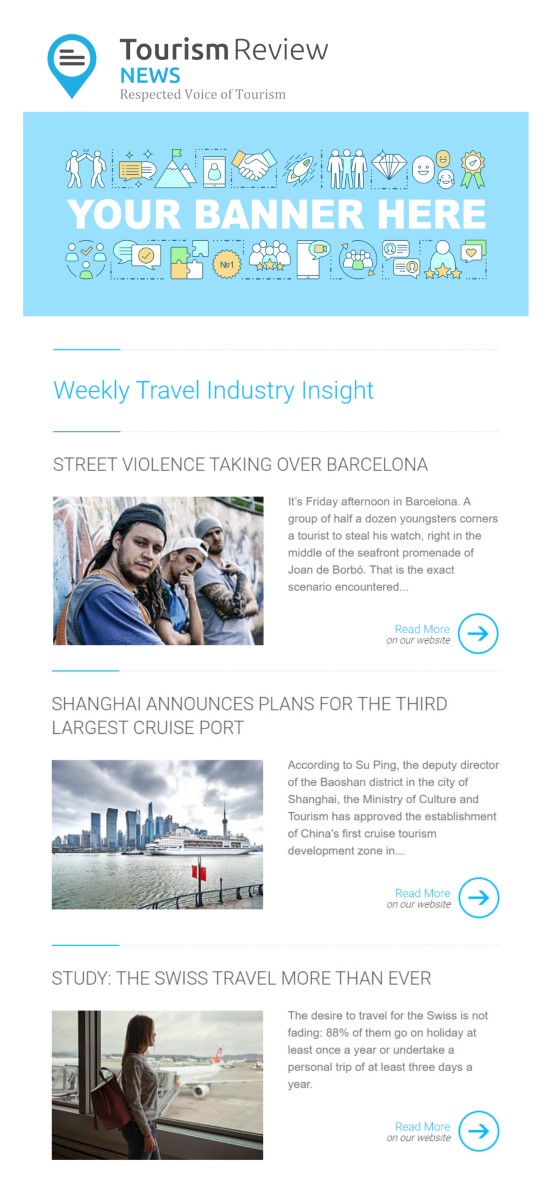This is a detailed smartphone screenshot of the Tourism Review News website. 

At the top of the image, there's a logo resembling a location pin, rendered in blue with a white circle in the center and three black lines.

Directly below this logo, the text reads, "Tourism Review News: Respected Voice of Tourism." Beneath this heading is a blue banner displaying the message "Your Banner Here."

Following this banner, the site header reads, "Weekly Travel Industry Insight," introducing the listed articles.

The first article is titled "Street Violence Taking Over Barcelona." The content describes an occurrence on a Friday afternoon in Barcelona where a group of six youngsters attacked a tourist to steal his watch on the seafront promenade of Joan de Bordeaux. Accompanying this article, there's an image presumed to show the so-called "thugs" involved in the street violence.

The second article is "Shanghai Announces Plans for the Third Largest Cruise Port." The image associated with this article depicts the city skyline as viewed from across a waterway.

The third article is "Study: The Swiss Travel More Than Ever," accompanied by an image featuring a woman gazing out of an airport window, overlooking the tarmac.

Each article preview is designed to provide quick insights into current events and trends within the travel industry, complemented by relevant images to enhance reader engagement.